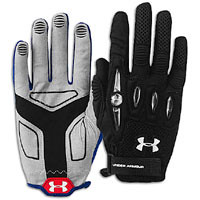The image features a pair of Under Armour gloves, displayed against a white background as if floating. The right glove is black with a white Under Armour logo and the words "Under Armour" in the bottom left corner. The left glove is a light gray with a dark gray Y-shaped pattern in the middle, featuring a red Under Armour logo with white lettering. The gloves are positioned to show both their front and back sides; the black glove displays the palm, while the gray glove shows the back. The overall presentation makes it appear almost like a digital rendering rather than a photograph.